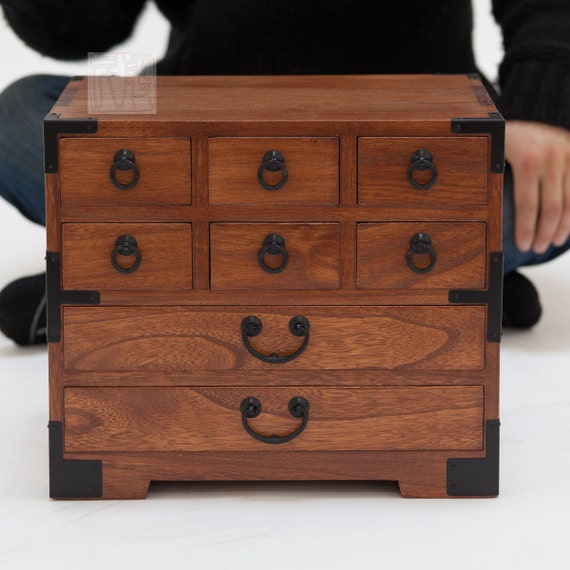In this image, a rectangular chest of drawers sits on a white floor as a partially visible person is positioned behind it. The chest is made of medium brown wood, darker than pine but lighter than cherry, and features black wrought iron accents. These accents include circular handles on each of the six small drawers at the top, situated in two rows of three, and half-circle handles on the two larger, full-length drawers at the bottom. The same black metal is found at the corners of the chest, likely providing both decorative and structural support. The chest appears to be around 10-12 inches tall and 12-14 inches wide, with small feet that slightly elevate it from the ground. 

Behind the chest, a person sits cross-legged, dressed in a black long-sleeve sweater and blue jeans. The photo reveals only the lower half of their body, focusing on their legs and the position of their hands. The person's left hand rests on their left knee, while their right elbow is bent, with the right hand out of the frame. Their black socks are visible against the white floor, adding to the high contrast of the scene. The overall composition centers the wooden chest, enhancing its detailed craftsmanship and rich wood grain against the stark background.